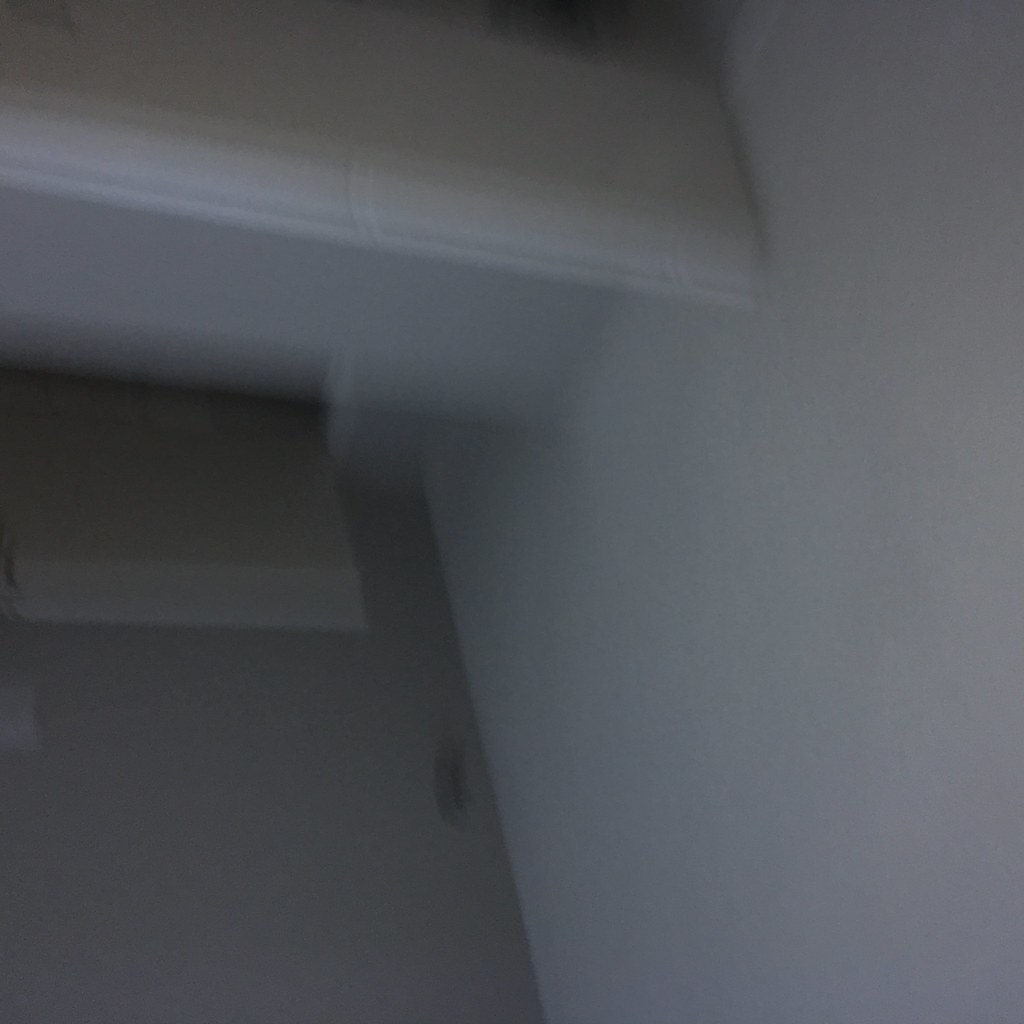The image depicts a very out-of-focus scene dominated by a primarily white object, which spans both the side and the back of the frame. The rear area of this object appears slightly darker, potentially due to shadows falling across it. In the top left corner, there is a long, rectangular shape featuring a pronounced lip at the top, where the upper edge extends outward further than the lower edge. This shape exhibits a textured surface. Attached to the bottom of this rectangular form is a smaller, square piece in a somewhat darker hue, extending downward. Additionally, there is a noticeable dark stain or scribble-like mark located towards the bottom of the frame.